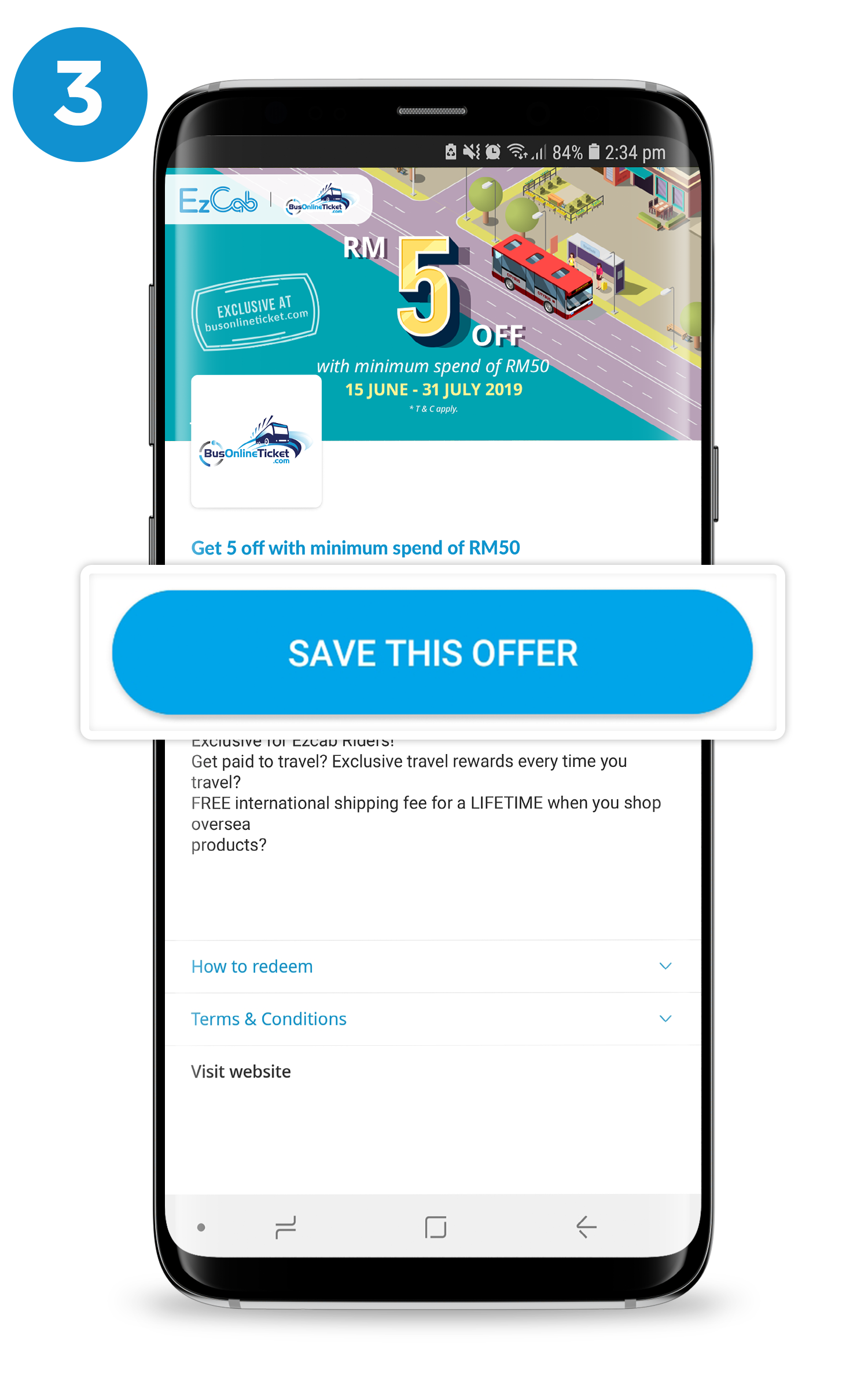This advertisement screenshot features a clean white background. In the upper left corner, a blue circle with white text displays the number "3". Dominating the center of the advertisement is a smartphone with black bezels. On the smartphone's screen, a prominent white pop-up menu appears as a white rectangle containing a blue oval button with white text that reads "Save This Offer".

At the top of the smartphone's screen, a black status bar is visible, displaying various icons including those for battery level, alarm, Wi-Fi, and mobile signal strength, along with the time, 2:34 p.m. Below this status bar, the main content on the phone screen features an endearing graphic of a pixel art bus on a road next to the ocean, stationed at a bus stop with two small trees nearby. 

On top of this image, in the upper left corner, there is a white rectangle with blue text that reads "Easy Cob". Next to this text is a faint logo that is difficult to discern. In the center of the smartphone's screen, bold text advertises the main offer: "RM5 Off with Minimum Spend of RM50," valid from 15 June to 31 July 2019. A repetitive statement underneath reaffirms the offer: "Get 5 Off with Minimum Spend of RM50."